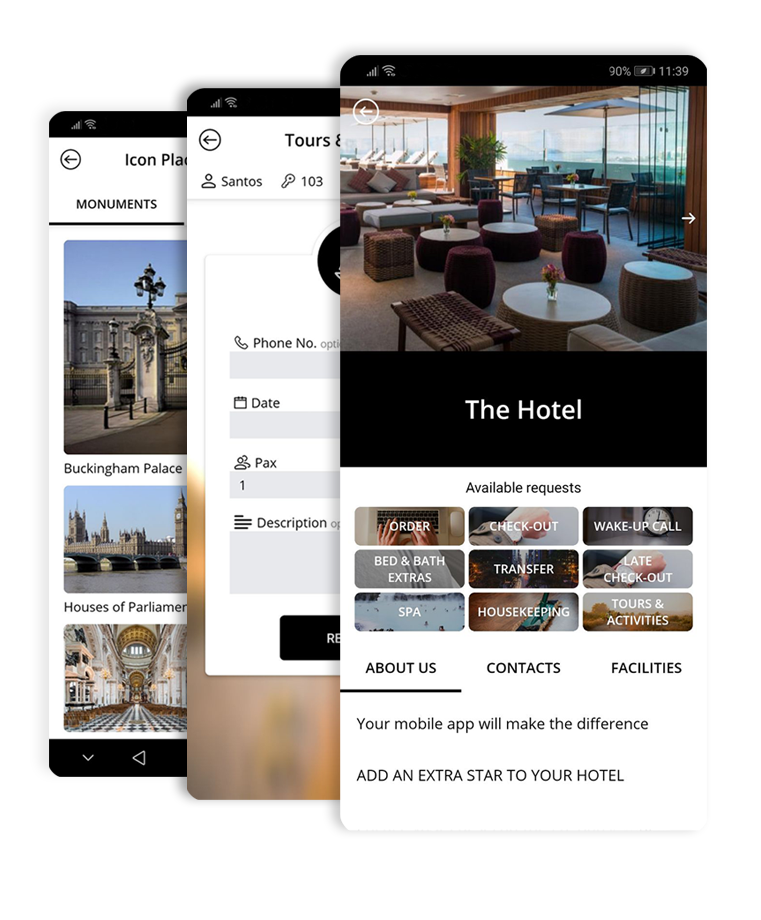An image depicts three stacked windows on a cell phone screen, with increasing size from left to right. The leftmost window, partially visible, features icons and monuments, including prominent exterior images of Buckingham Palace and the Houses of Parliament. Buckingham Palace is characterized by its grand stone architecture, columns, and front gates. The Houses of Parliament window contains a view of a bridge over a river, with Big Ben on the right and a historic building with tiered spires. At the bottom, an interior view of a historic church with a central dome is partially visible.

The middle window, also partially visible, focuses on tour information with an icon of a small person labeled "Santos" and the number "103" next to a down-facing key symbol. Options for inserting a phone number, date, PAX, and a description are available.

The rightmost and fully visible window showcases the interior of a hotel common area, identified by a black banner with white text reading "The Hotel" in the center of the page. The hotel interior includes a couch, several round tables with small flower arrangements on about a third of them, and barrel-shaped purple cushioned chairs. In the foreground, there's additional seating made of brown woven material. To the right, an umbrella and chairs on a terrace can be seen, and the background features what appears to be loungers around a pool.